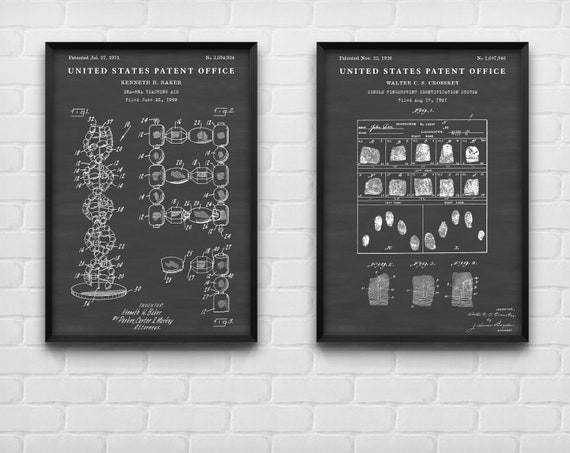The image displays two detailed charts, side by side, mounted on a white brick wall. Both charts, measuring approximately 4.5 inches wide by 6 inches tall, bear the header "United States Patent Office" in white text on a dark background, positioned about half an inch from the top. They are spaced roughly an inch apart.

The chart on the left features a patent attributed to someone named Kenneth H. Baker. It has a date, difficult to read, in the upper left corner, potentially indicating July 17, 1903. The central illustration depicts intricate circular structures, starting with larger circles composed of smaller circles, suggesting a scientific or structural diagram, possibly a helix or molecular chains. The right side of this chart contains various barrel-shaped objects, adding to the complex technical design.

The right chart credits Walter Cressley, Cresskey, or a similarly hard-to-read name. Dated March 1930-something, it includes numerous small squares aligned in rows, resembling fingerprint patterns or possibly photographs of granular objects like rocks or gems. Below these squares, two larger squares display images resembling footprints or handprints, with more at the bottom in gray, all extensively labeled though illegible. Each element of these patents shows the meticulous detail required for such documentation, presenting a fascinating glimpse into historical patent filings.